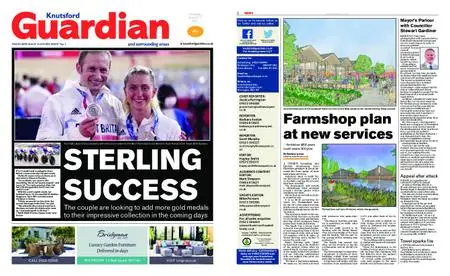In the image, we see two distinct newspaper pages laid out side by side. The left page is filled with small text, but a larger headline in the lower left corner reads "Nutzford" in blue text, accompanied by "Guardian" in large red text. Below this headline is a photograph featuring a young man and woman, both likely in their early 20s, who are proudly wearing blue lanyards and medals. They are dressed in white jackets with blue and red accents. The man, positioned on the left, sports an Adidas logo on his jacket and is smiling while holding his medal in his right hand. Beneath the photo, against a black background, a bold white headline states "Sterling Success," indicating that the couple plans to add more gold medals to their impressive collection in the coming days. On the adjacent page, another article features a bold black headline that reads "Farm Shop Plan and New Services."